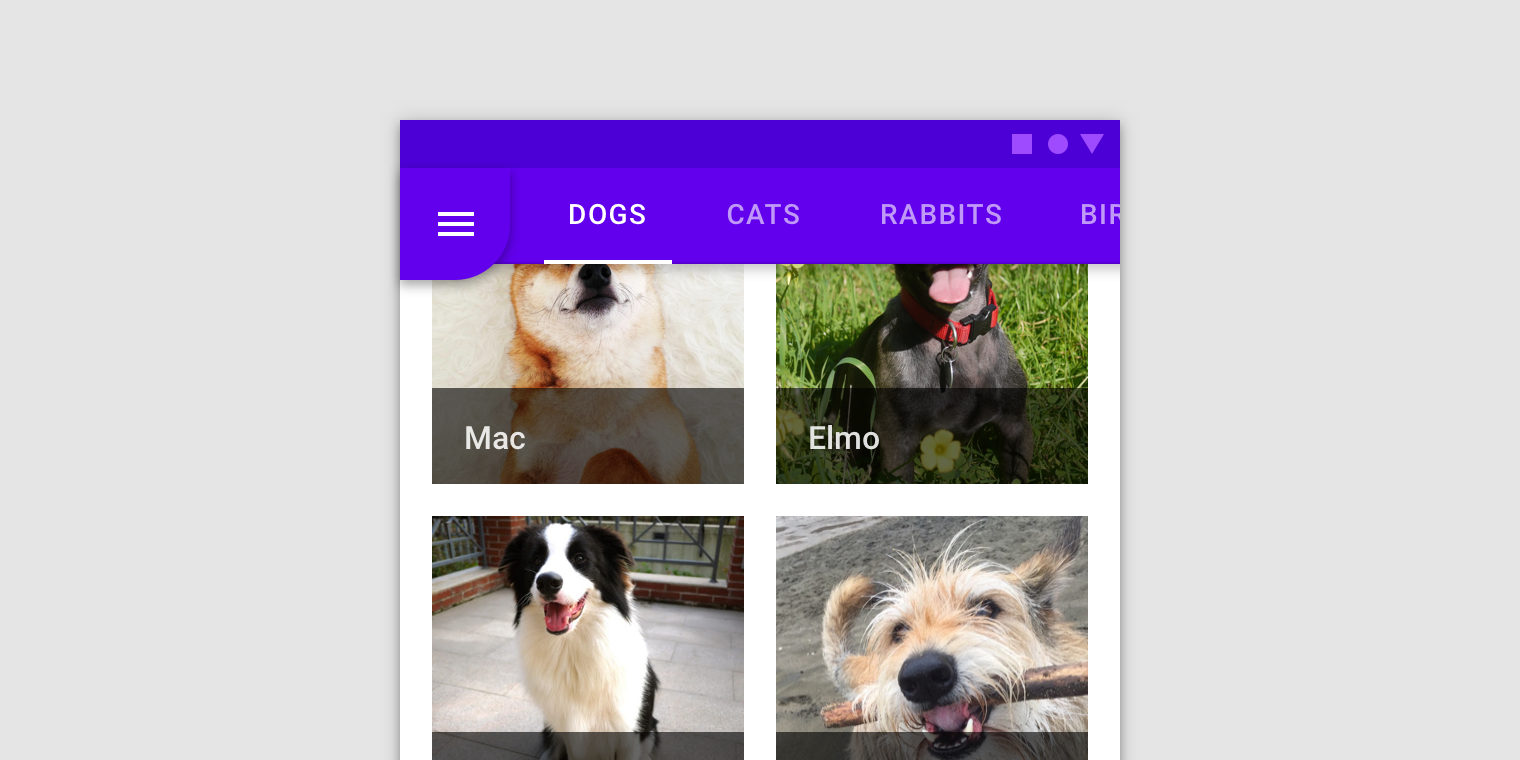This cropped screenshot captures a section of the mobile version or a mock-up of the Petfinder.com website. In the top-right corner, there is a cluster of icons—a square, a circle, and an upside-down triangle—all in a light shade of purple. At the left of these icons, a white menu icon can be seen. Beneath this cluster, a horizontal list of categories is displayed: "Dogs," "Cats," "Rabbits," and "Birds," although the last two letters of "Birds" are cropped out.

Directly below this menu, the partial view of four individual animal listings is visible. Each listing is in a square format with a photo of the animal at the top and a light black bar at the bottom displaying the animal’s name in white text. The first animal appears to be a Shiba Inu laying on its back, although its head is cropped out of the image; this animal is named Mac. To the right of Mac, there is a black dog named Elmo. The bottom two animal photos are also partially cut off, showing only the upper halves of their images.

The entire screenshot is set against an oversized gray background, creating a large rectangular gray box with the cropped screenshot of the app centered within it. Large empty spaces are visible to the left and right of the image, as well as above and below it.